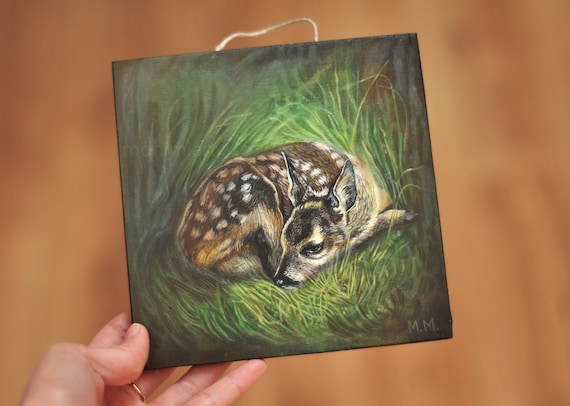The image displays a small, square painting, approximately 9 inches by 9 inches, held up by a woman’s left hand adorned with a thin ring band on her middle finger. The painting features a detailed depiction of a young fawn, curled up and resting peacefully in a nest of green grass. The fawn, characterized by its brown fur and distinctive white spots, has a life-like quality thanks to the artist's use of light to illuminate the animal, creating a sense of depth and realism. The surrounding grass is rendered with more detail near the fawn, gradually becoming less distinct and darker as it extends upward, accentuating the central focus on the baby deer. The background where the painting is being held features a brown-orange undertone, enhancing the warmth of the scene. At the top of the painting, a small white string allows for easy hanging, and the artist’s initials "MM" are subtly marked at the bottom of the canvas.